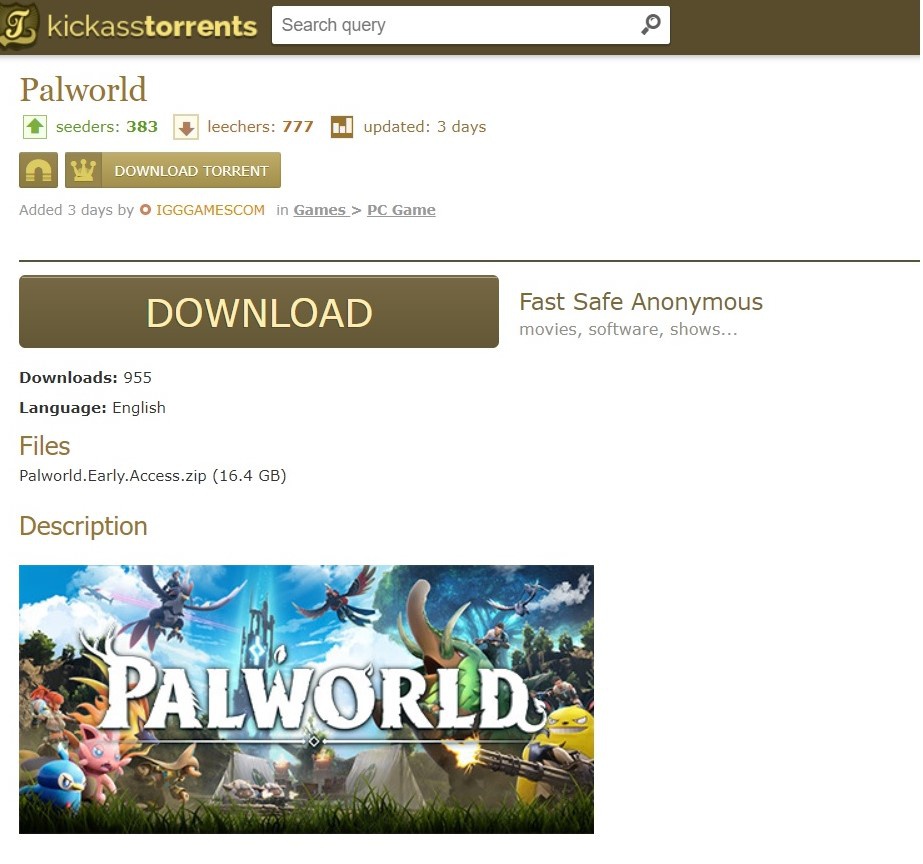This screenshot captures a square-oriented interface on the Kick-Ass Torrents website, identified by its distinct dark brown top banner. The banner features the "Kick-Ass Torrents" logo and stylized text, with "Torrents" in bold yellow font. To the right, there's a white search box accompanied by a magnifying glass icon.

Beneath the banner in brown text is the title "Powell World," followed by various control icons and status indicators. These include an upward arrow with "Cedars 383," a downward arrow labeled "Leachers 777," and a graph icon indicating an update three days ago.

Lower down, a row of icons including a magnet, a crown, and a "Download Torrent" button is visible, along with the addition note: "Added 3 days ago by IGGGAMESCOM in games / PC game." Below this row, a thin brown line separates sections of the interface.

Prominently featured is a large brown "Download" button with the text "Fast, Safe, Anonymous" to its right. Directly under this button, it states "955 downloads" and specifies the download language as English. Sections showing file information and description details follow.

At the bottom left corner of the image, there is an illustration of the game "Powell World," marked by large white text of the same title. This segment stands out against a contrasting white empty space to the right.